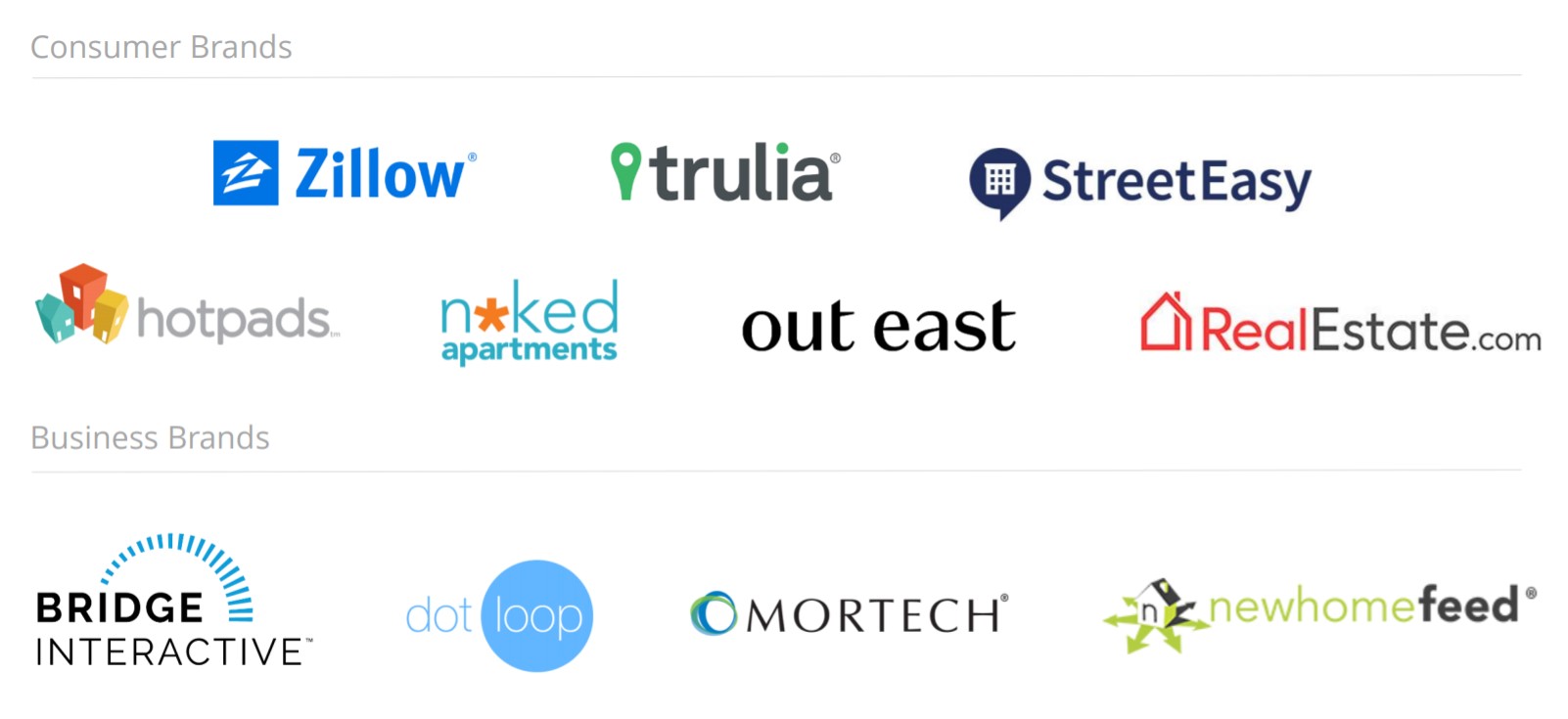The image is a computer screenshot displaying a collection of various brand names and their logos against a white background. At the top left corner, the heading "Consumer Brands" is written in light gray text, underlined by a light gray line that runs horizontally across the image.

The first row from the top features the following logos and names:
1. Zillow: A blue square with a house symbol featuring a "Z" inside it, with "Zillow" in blue text.
2. Trulia: A green pin icon resembling a location marker, accompanied by "Trulia" in black text.
3. StreetEasy: A speech bubble icon incorporating a map design, with "StreetEasy" written in blue or black text.

In the second row:
4. HotPads: An arrangement of green, orange, and yellow buildings as the logo, with "HotPads" written next to it.
5. Naked Apartments: A logo primarily in blue, with an orange star used in place of the "A" in "Apartments."
6. Out East: The text "Out East" in black, with a little red house followed by "realestate.com" in black text.

The third row includes:
7. Bridge Interactive: A blue arc symbolizing a bridge, with "Bridge Interactive" written alongside it.
8. DotLoop: A logo featuring a blue dot behind the word "loop."
9. Mortech: An emblem composed of circular symbols, located to the left of the brand name "Mortech."
10. New Home Feed: A small house icon with green and black arrows, with the text "New Home Feed" written next to it.

The entire image is set on a plain white background, presenting a clean and organized display of the consumer brands and their respective logos.